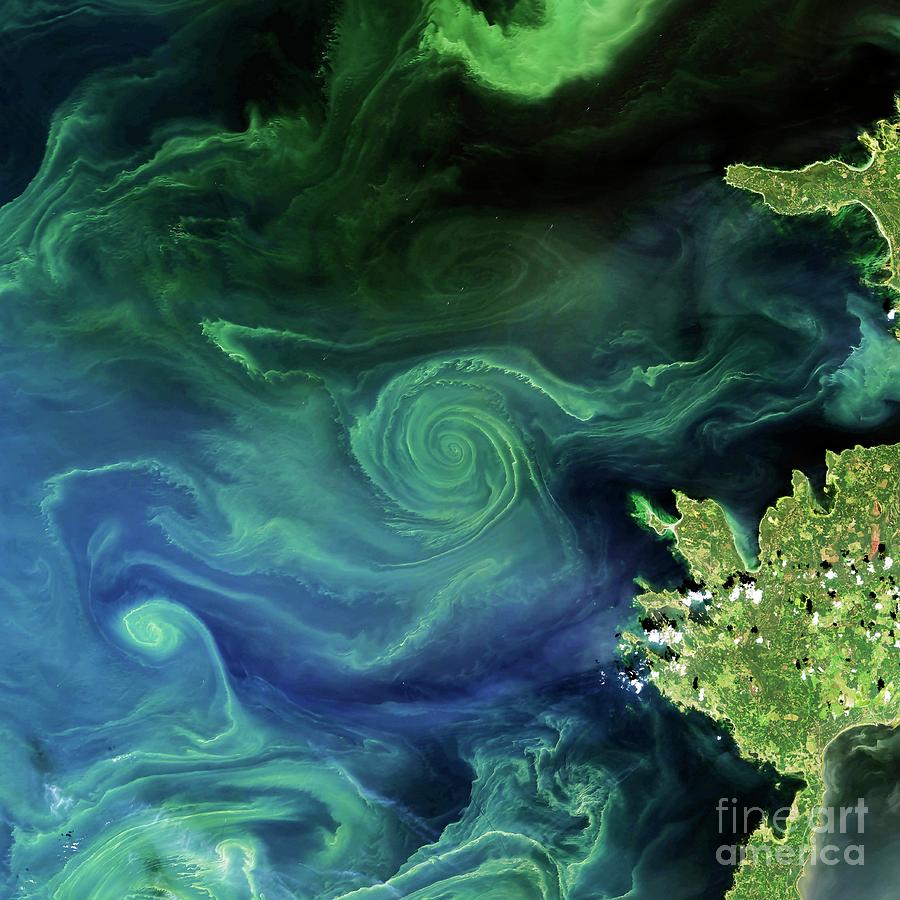This satellite image captures an aerial view of the ocean, highlighting bioluminescent swirls of vibrant green against a backdrop of deep blue waters. The waves create dynamic, circular, and typical motions throughout the scene. To the left, a small landmass is visible, topped with hovering white clouds, while to the right, there is another landmass, slightly larger, where you can discern the tops of some buildings or structures. Despite the abstract nature of the bioluminescent patterns, the details of the land and atmospheric elements ground the image in reality. This captivating image also features a transparent "Fine Art America" watermark in its bottom right corner.